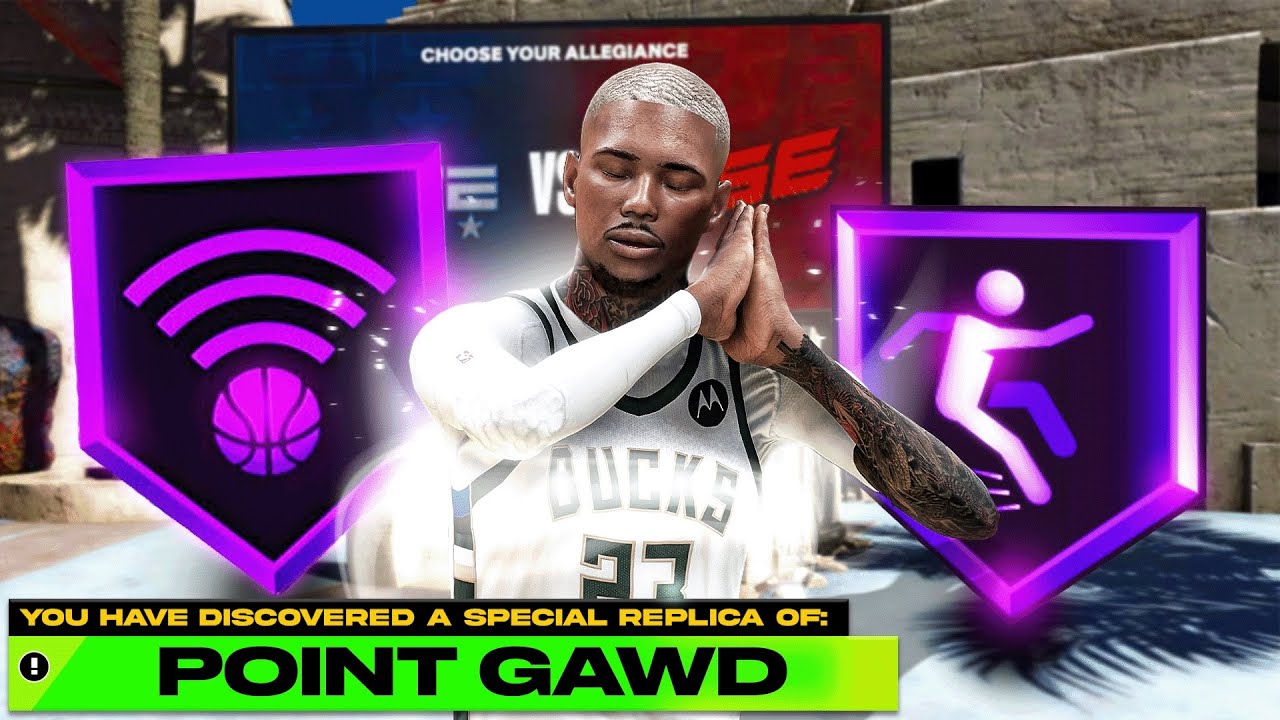In the photograph, an NBA player is prominently displayed wearing a Milwaukee Bucks jersey with the number 23. His eyes are closed, and his hands are positioned near his ears, reminiscent of a "go to sleep" gesture. The jersey appears to be the Bucks' home uniform, characterized by its white fabric and green lettering.

On either side of the player, two emblematic designs are visible, each shaped like a baseball home plate. The design on the left features a purple border encasing a purple basketball. The one on the right mirrors this style but includes a figure that appears to be in motion, although the details are indistinct.

The lower left corner of the image has a segment of black background with yellow text that reads, "You have discovered a special replica of". Adjoining this text is a green background with black lettering that includes the phrase "point called with God," spelled uniquely as G-A-W-D. Behind the player, the scene includes the outline of a building and some trees, adding depth to the background. The overall composition combines elements of sports memorabilia and dynamic athletic portraiture.